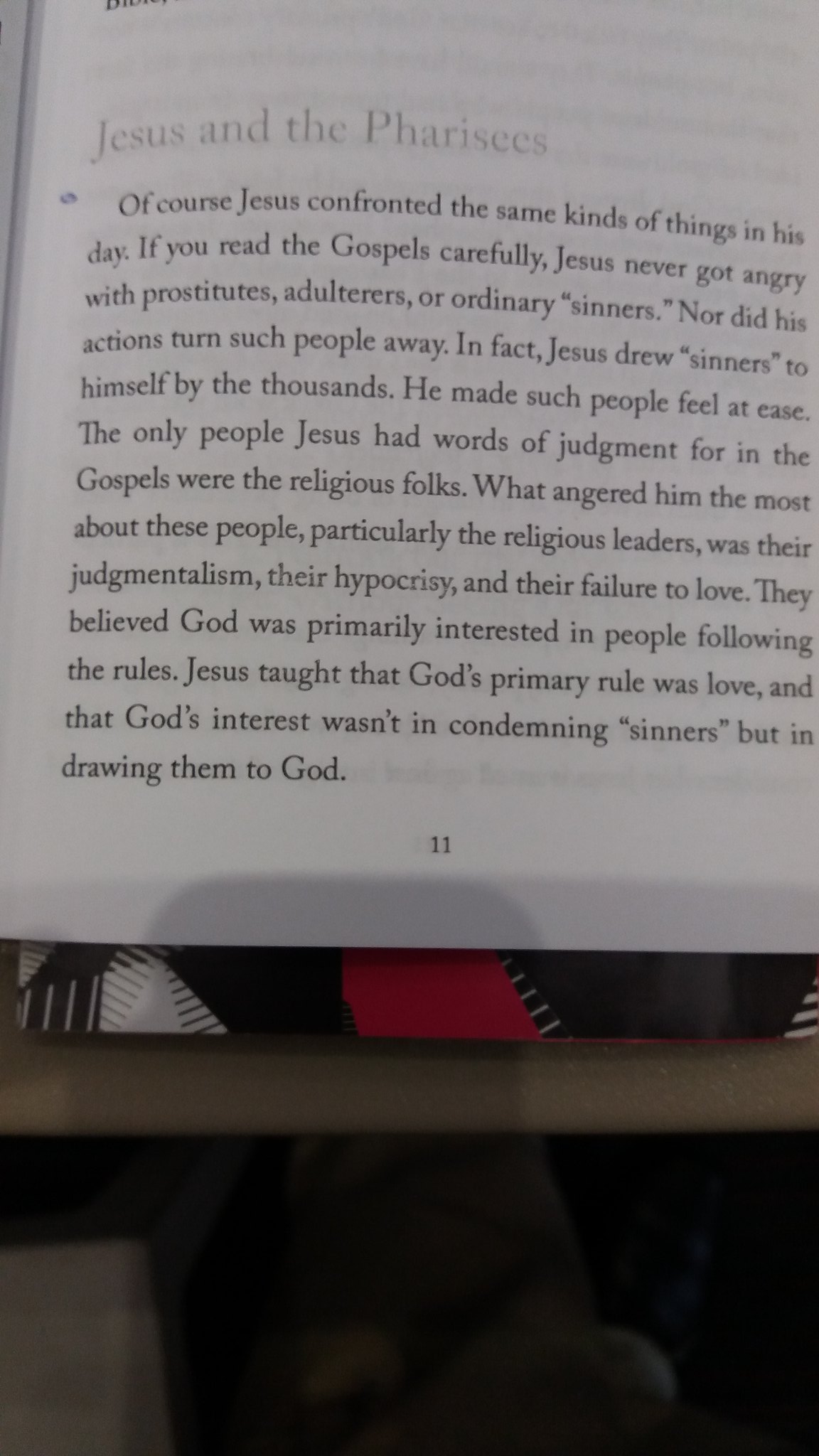This image captures a close-up of the lower half of page 11 from a book, displaying text under the subheading "Jesus and the Pharisees." The detailed excerpt explains how Jesus, during his time, never demonstrated anger towards prostitutes, adulterers, or ordinary sinners, but rather drew them to him by the thousands, making them feel at ease. The only people he judged were the religious leaders, criticized for their judgmentalism, hypocrisy, and lack of love. The text emphasizes Jesus's teaching that God's primary rule is love, contrary to the religious leaders' belief that God was mainly concerned with rule-following. The page is set against a background that includes blue, red, and black elements, possibly indicating a lap desk or table. The visible colors in the image are gray, white, black, red, and tan, suggesting a subdued yet varied palette.